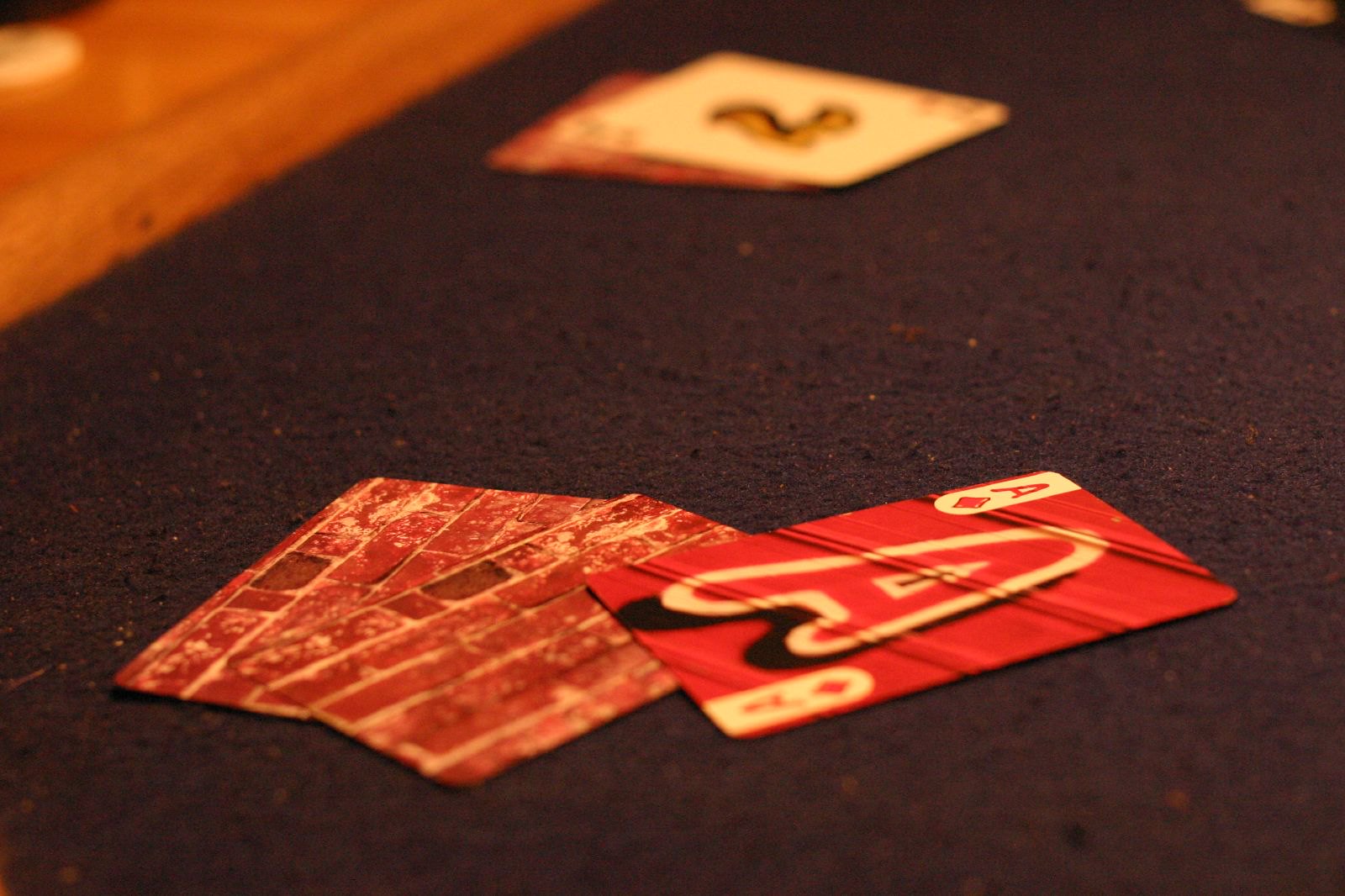This detailed caption could be used to accurately describe the image:

"In this close-up, square image, we see a collection of playing cards arranged on a blue felt-covered table, which shows signs of wear with small snags and fabric balls. At the center of the composition, two playing cards are face down, featuring a design that mimics a brick wall. The first of these cards is positioned vertically, while the second card lies at an angle to the right, its left corner overlapping the bottom card. Resting atop this arrangement is a red Ace of Diamonds card, also angled to the right. The Ace is adorned with a large 'A' in the center, outlined in white, and a diamond symbol along with the 'A' in the top-left and top-right corners. In the background, the light-colored wooden side rails of the table can be seen, albeit blurred. Additionally, there's a partially visible, blurry image of two more cards; one is face down and the other, angled and face up, displaying a yellow number seven on a white surface."